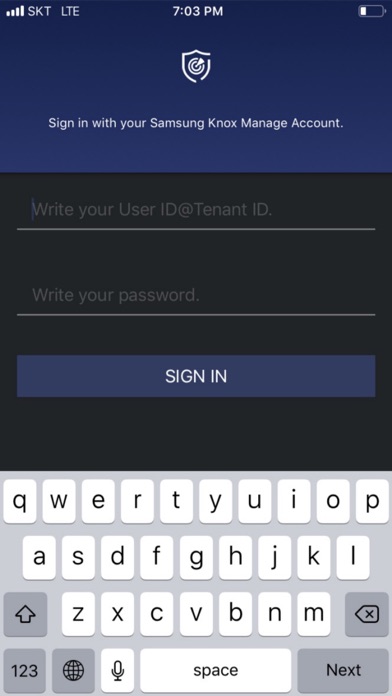The image depicts a smartphone screen displaying a login page for managing a Samsung Note account. The top portion of the page features a blue background with white text reading "Sign in with your Samsung Note manage account." Above this text, there is a white shield icon with two concentric circles in the center and an arrow pointing towards the inner circle. 

Below the text, the page background shifts to black. The first text box, with a gray placeholder text stating "Write your user ID or tenant ID," currently has a cursor placed inside it. The second text box is designated for entering the user's password and also has gray placeholder text saying "Write your password."

Further down, there's a prominent "Sign in" button with white text set against a blue background. At the bottom of the screen, the smartphone's virtual keyboard is visible. The keyboard has a gray background, white keycaps with black letters, and specific function keys—such as the Shift, Number, Language, Next, and Back buttons—which are all gray.

The overall layout is user-friendly, guiding users step-by-step to sign in with their Samsung credentials.